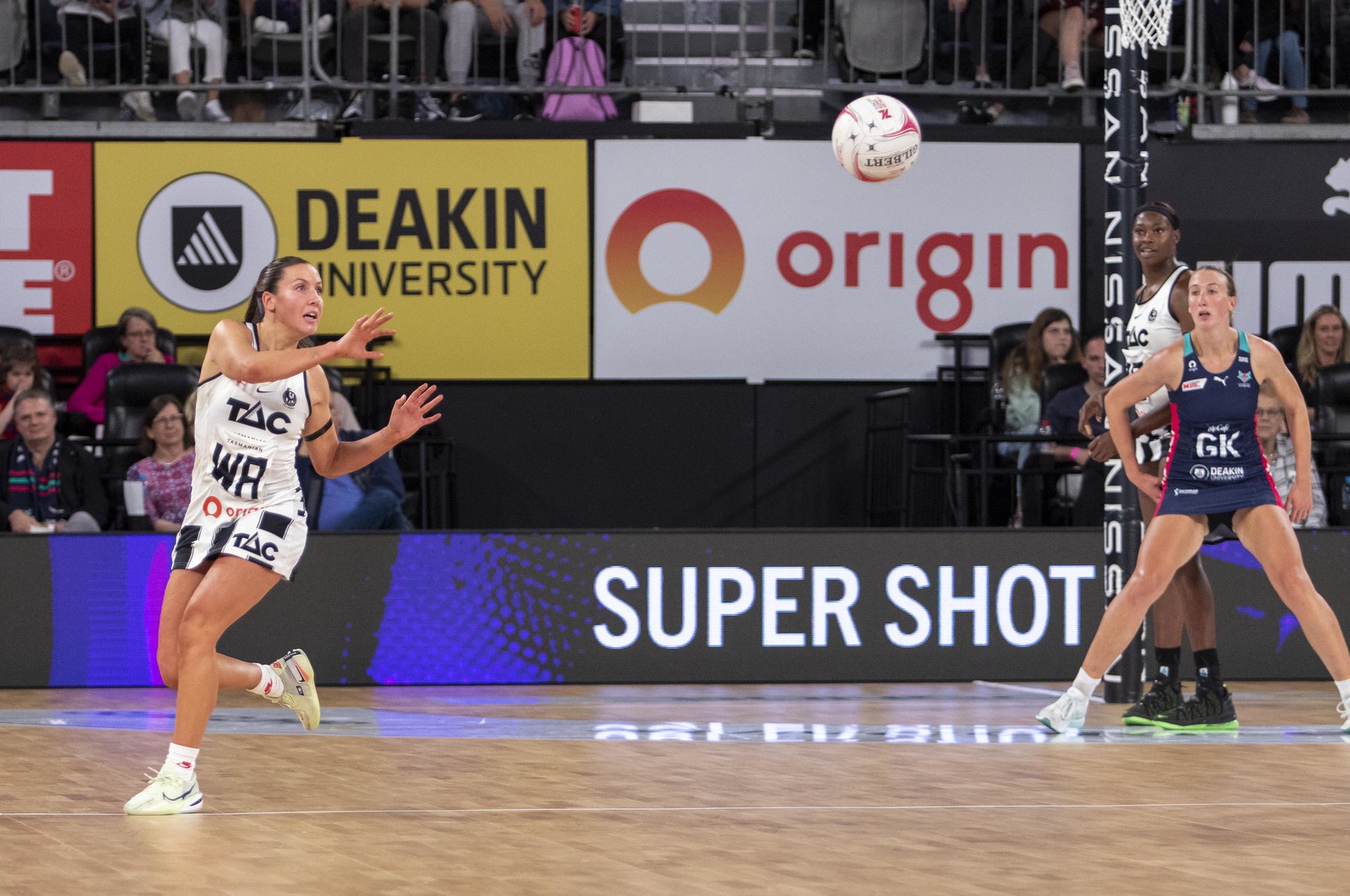In the image of a basketball game on an indoor court, we see three female players intensely engaged. The player in the dark blue and red outfit with the initials 'GK' stands centrally, poised with a ball arcing towards her from the upper part of the picture. This ball is distinctive, white with red lines and some black text. The player receiving the pass sports a white and black jersey, her hands outstretched in anticipation, wearing white tennis shoes. Positioned slightly behind and above her is a taller woman, also in a white and black outfit with black socks and shoes, possibly indicating the league’s team colors.

The court's polished wooden floor reflects the indoor lighting and parts of the text "Super Shot," prominently displayed in white capital letters on a banner at the arena's lower wall. The background reveals a section populated by spectators, who are seated both in the lower bleachers close to the court and the upper stands. Advertisements can be seen behind the crowd, including a yellow banner for Deakin University, a red and orange circular logo for Origin, and a Puma ad on the right side. The atmosphere is vibrant with a diverse mix of colors from the spectators' attire and the arena decor, including spots of black, white, orange, yellow, dark blue, and purple. In the upper deck, a hint of a pink-clad figure suggests the presence of a young child among the viewers.